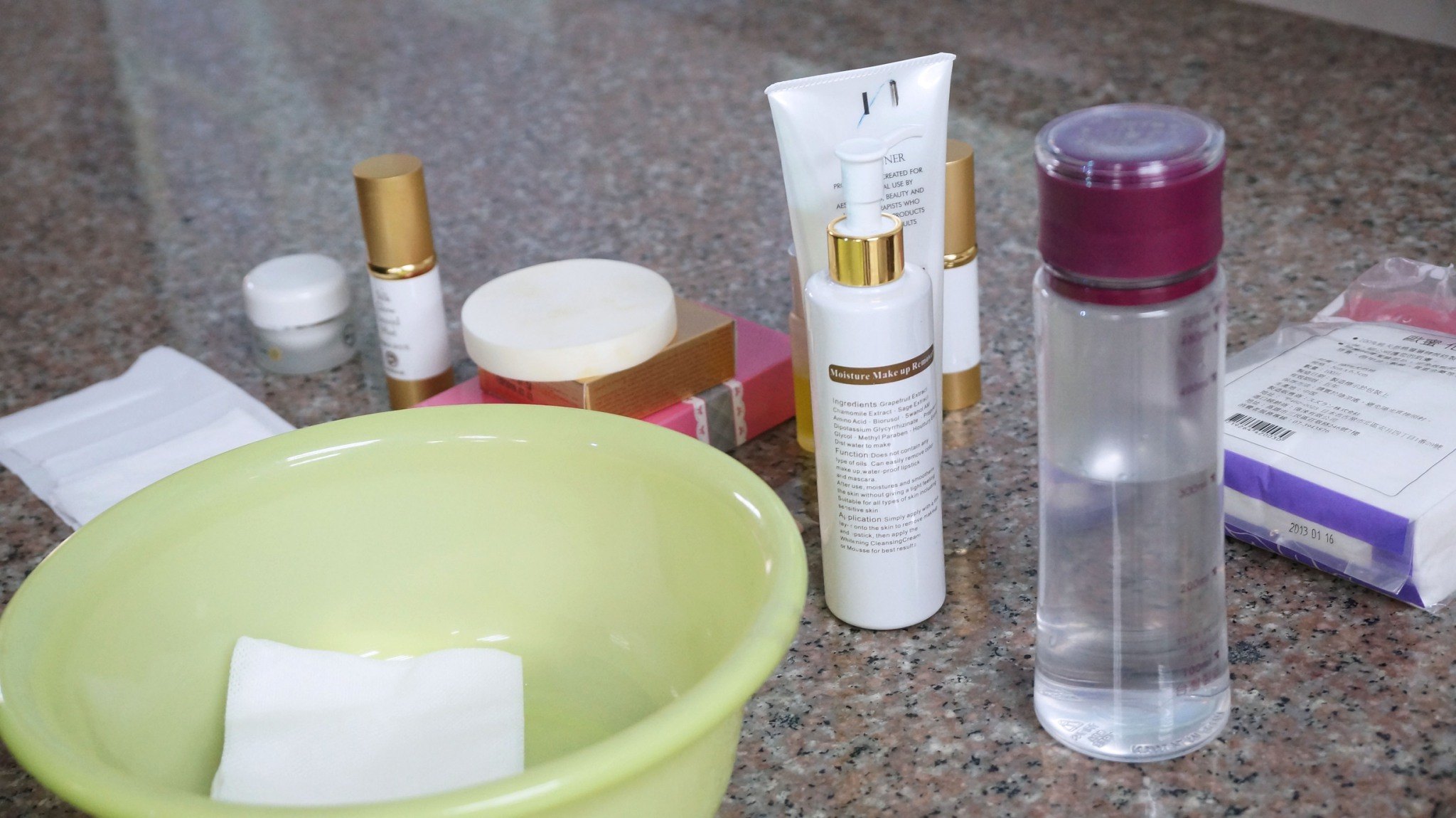In this detailed photograph of a marble countertop, likely set in a kitchen or bathroom, the surface showcases a visually captivating blend of orange, pink, black, and white hues. Arranged neatly on the counter are various skincare products, suggesting a setup for a home spa day. 

In the lower left corner, a large lime green bowl holds a white facial wipe. Centered among the other items, two boxes stand out: the upper box is gold, while the lower one is pink, adorned with a blue lacy ribbon tied around its center. Surrounding these boxes are multiple tubes and containers dedicated to skincare, including a container of lotion and several spray bottles.

To the right, a prominent clear container filled with a transparent liquid is capped with a burgundy or magenta lid. Further right, a package of what seems to be facial wipes or cleansers completes the arrangement, adding to the impression of a thorough and well-organized skincare routine.